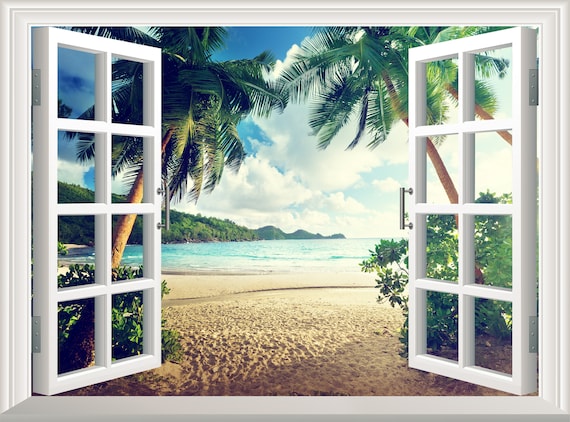The image depicts an artistic representation resembling a white-framed French window opening out from the center, featuring two window doors adorned with metallic handles. The window's design is detailed with slats forming eight square panes, and the entire frame is immaculately white. Through the open windows, a picturesque tropical beach scene unfolds, showcasing white-yellowish sand and turquoise water. On either side of the window, palm trees or coconut trees lean inward, framing views of lush green hills or mountains in the distance. The sky is a mix of clear blue with patches of white clouds, and sunlight bathes the entire landscape, casting a serene and warm atmosphere.